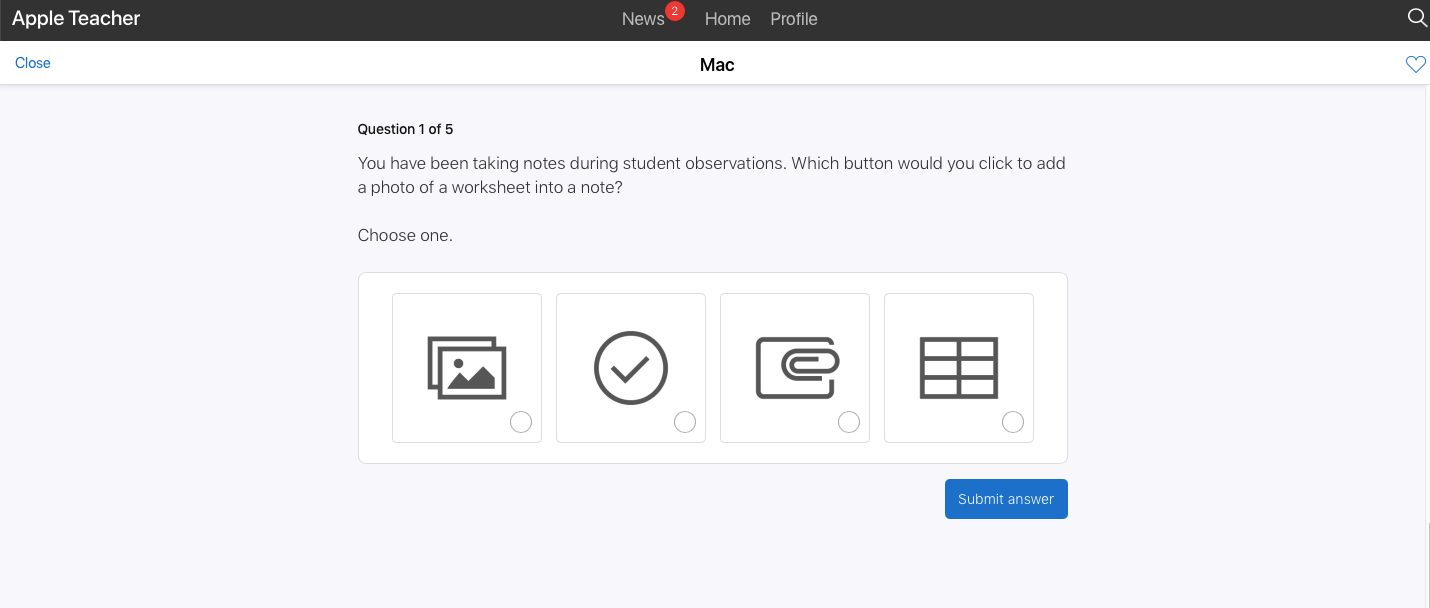The image features a light blue background with a long black bar at the top displaying the text "Apple Teacher" in white letters. Additionally, this bar includes icons for "News" (highlighted with a red circle containing the number 2), "Home", and "Profile", as well as a magnifying glass icon on the far right.

Below the bar, there is a white box with the Apple logo in blue, the word "Mac" in the middle, and a small blue heart icon on the right.

Further down, the blue background continues and presents the text "Question 1 of 5." The text explains: "You have been taking notes during student observations. Which button would you click to add a photo of a worksheet into a note? Choose one."

Beneath this explanation, there is a large white box containing four smaller boxes, each with a circular radio button for selection. The first box features an icon of two pages with an image resembling black mountains and a black sun. The second box displays a black circle with a checkmark inside. The third box shows a paperclip attached to a piece of paper. The fourth box has a grid icon divided in half horizontally and into thirds vertically, resulting in six smaller boxes overall.

Below these options, there is a blue button labeled "Submit Answer."